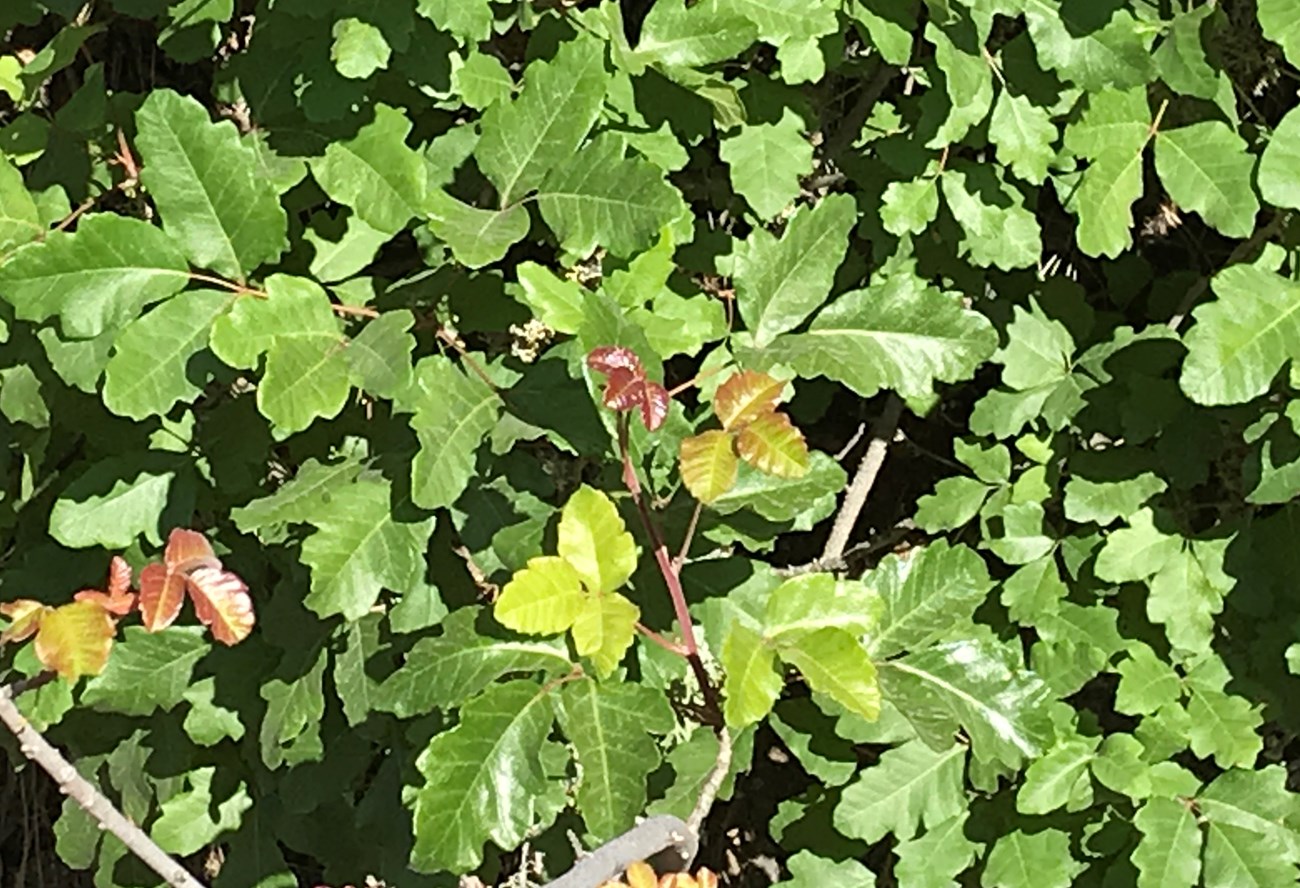The image captures a bright, sunlit outdoor scene densely packed with green foliage. It appears to be either an assortment of young tree seedlings or the dense leaves of a mature shrub or tree. There is a mix of various shades of green, with the newer leaves tinged with lighter greens and dark reds, transitioning to the larger, deeper green leaves. Some leaves are arranged in a three-part composition reminiscent of a fleur-de-lis. The lighting is vivid, casting noticeable shadows of leaves upon one another, accentuating the texture and detail. Among the green, a few leaves exhibit hues of red and orange, suggesting the early stages of color change. Scattered throughout the foliage are visible branches and stems, with no other discernible items or insects present in the image. The intricate, close-up view highlights the diverse forms and colors of the leaves, creating a rich tapestry of natural beauty.